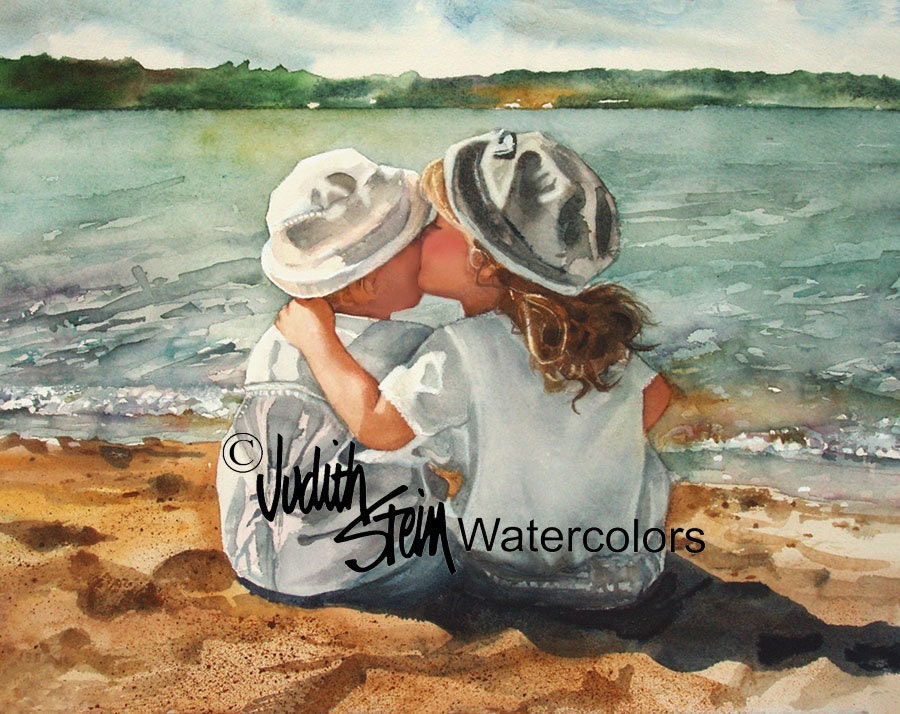Title: "Childhood Serenity by the Shore"

Description: This detailed watercolor painting captures a tender moment of two children sitting together on a sandy beach, their gaze fixed on the serene waters ahead. The child on the left, possibly a boy, and the child on the right, a girl with long blonde hair, are both adorned in white attire – possibly t-shirts or light jackets – complemented by hats shielding them from the sun. Their lower clothing remains indistinguishable, concealed by their seated posture in the sand. The scene is beautifully bathed in sunlight, casting soft shadows that stretch across the sandy expanse, which dominates the mid to lower section of the painting.

In the background, the calm, shallow waters of the ocean gently lap at the shore, rendered with exquisite watercolor technique that adds a dreamy quality to the scene. Farther back, blurred greenery hints at distant trees, merging subtly into the horizon. The sky is a delightful wash of blue, dotted with fluffy white clouds that add to the painting's tranquil ambiance.

The artwork bears the signature of Judas Stein, complete with a copyright symbol, subtly inscribed in black ink over the backs of the children, adding an element of authenticity to the piece. This painting beautifully encapsulates the innocence and simplicity of childhood, set against the timeless beauty of nature.